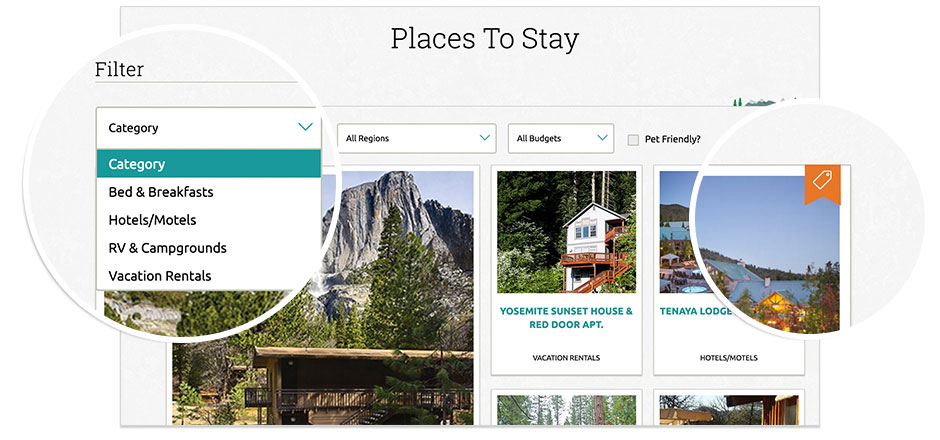The image features a gray background with a prominent header that reads "Places to Stay" in large black text at the top. Below the header are drop-down menus for filtering options labeled "Category," "All Regions," and "All Budgets," along with a checkbox to indicate if pet-friendly accommodations are preferred.

Beneath these menus, the image showcases three color photographs. The largest photo on the left depicts a picturesque cabin with a mountain in the background. To the right of this, a white house nestled against a lush forest backdrop is displayed, and the far-right image, partially obscured, appears to be a lodge.

Additionally, two magnified circular insets highlight specific details within the image. The larger circle on the left magnifies the "Filter" options, clarifying categories such as Bed and Breakfast, Hotels, Motels, RV and Campgrounds, and Vacation Rentals. On the right, a smaller circular inset magnifies a corner of one of the photos, revealing an orange banner that indicates the accommodation has been bookmarked.